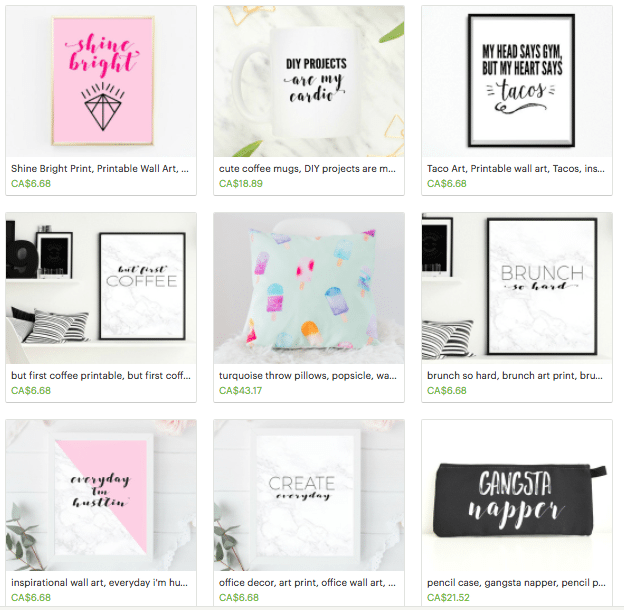This image is a neatly arranged screenshot showcasing a grid of nine items for sale, organized into three rows and three columns. Each item is displayed against its own background, enhancing the visual appeal.

**First Row:**
- **Top Left:** A product with a cream-colored background featuring the phrase "Shine bright like a diamond" in the center. Below this phrase, it reads "Shine bright print printable wall art" with a price tag of CA $6.68.
- **Top Center:** A coffee mug set against a marbled white background bearing the slogan "DIY projects are my cardio." It is described as "Cute coffee mugs, DIY projects" and is priced at CA $18.89.
- **Top Right:** This item shows a black-framed art piece with a white background that says "My head says gym but my heart says tacos." It is labeled as "Taco art, printable wall art, tacos" and costs CA $6.68.

**Second Row:**
- **Middle Left:** The scene depicts a room with a cream-colored background. In the upper left of the image, there's a shelf. Among the items displayed are some pillows and a framed wall art piece that reads "But first coffee." This piece is described as "Printable wall art," priced at CA $6.68.
- **Middle Center:** A pillow with a turquoise background, featuring popsicle designs. The description reads "Turquoise throw pillows" and is priced at CA $43.17.
- **Middle Right:** Another framed wall art print with a similar room setting and a cream background. This one says "Brunch so hard" and is listed as "Printable wall art" for CA $6.68.

**Third Row:**
- **Bottom Left:** A printable wall art piece with the phrase "Every day I'm hustling."
- **Bottom Center:** Another printable wall art piece that reads "Create every day."
- **Bottom Right:** The final item displays the phrase "Gangsta rapper" and is presumably another piece of printable wall art.

Each item is artistically captured, making it easier for potential buyers to visualize the products in their own spaces. Prices are clearly stated, providing an easy shopping experience.